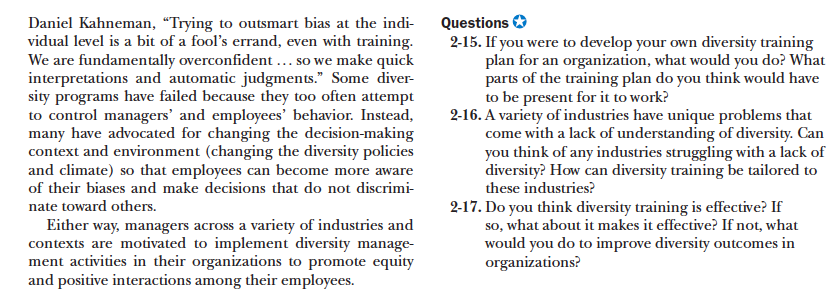This image is a screenshot, likely taken from a textbook or instructional manual. The text is presented in a uniform, serifed black font. On the left side, there are two paragraphs, including a quote from Daniel Kahneman. On the right side, there are a series of questions printed in black text, each accompanied by a blue circle featuring a white star. At the bottom of the image, there is the text "2-15" and the phrase "Thank you for watching!"